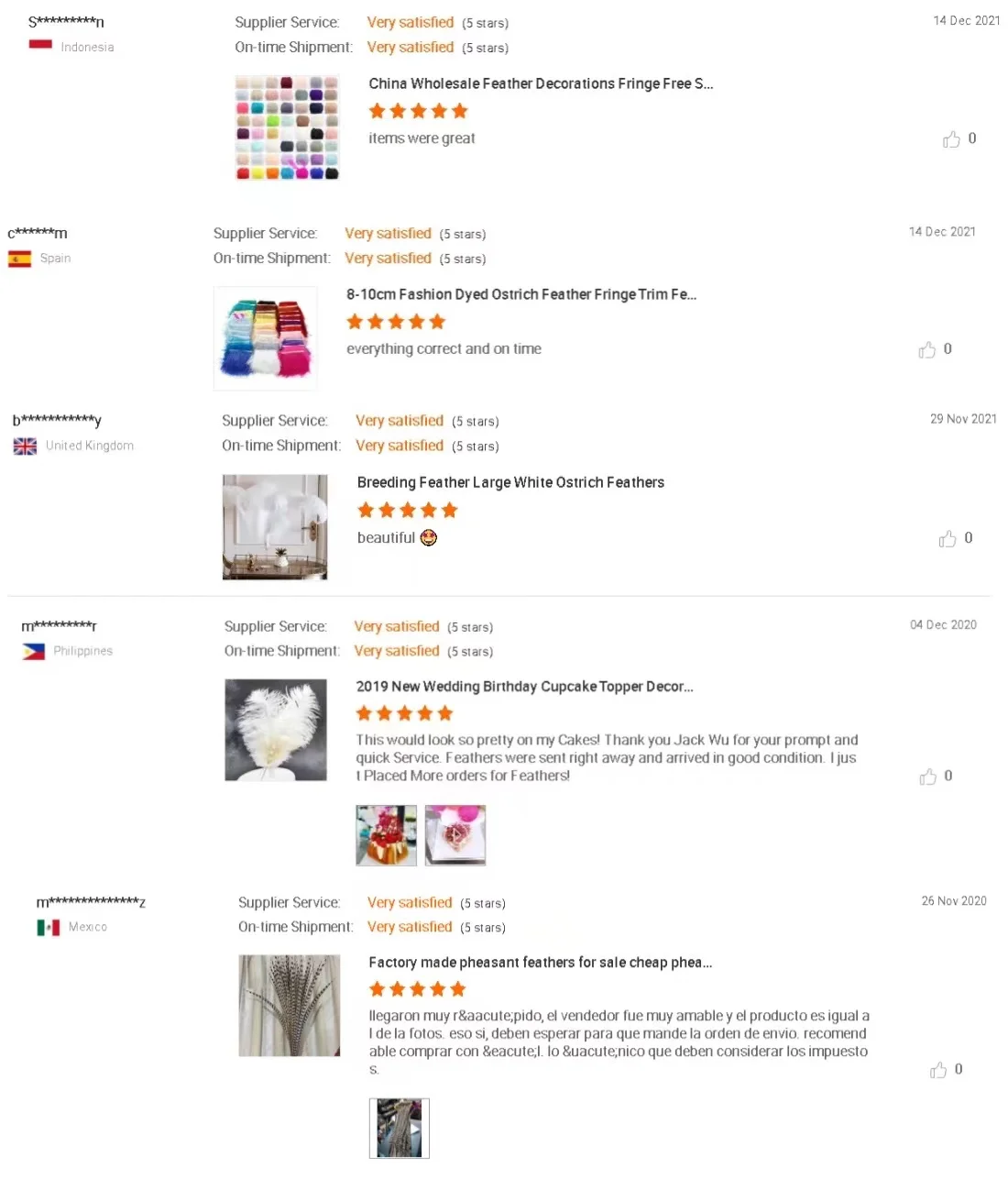This screenshot depicts an e-commerce wholesale platform interface, albeit highly zoomed out, making text readability challenging. The background is predominantly white. On the left-hand side, a column lists partially obscured usernames represented with initial and final letters followed by asterisks, along with their corresponding country flags. The countries featured include Indonesia, Spain, the United Kingdom, the Philippines, and Mexico. Adjacent to this column are images of various products available for purchase.

Just to the right, there is a column displaying service ratings for suppliers, including on-time shipment statistics and customer satisfaction scores. The assortment of products visible includes multiple types of decorative feathers such as colorful feather blocks, ostrich feathers, and factory-manufactured pheasant feathers. There are also items like birthday cake toppers. A text snippet indicates these products are listed under "China wholesale feather decorations fringe free," suggesting a focus on bulk purchasing options for decorative items. Overall, it appears to be a platform for sourcing wholesale decor items.